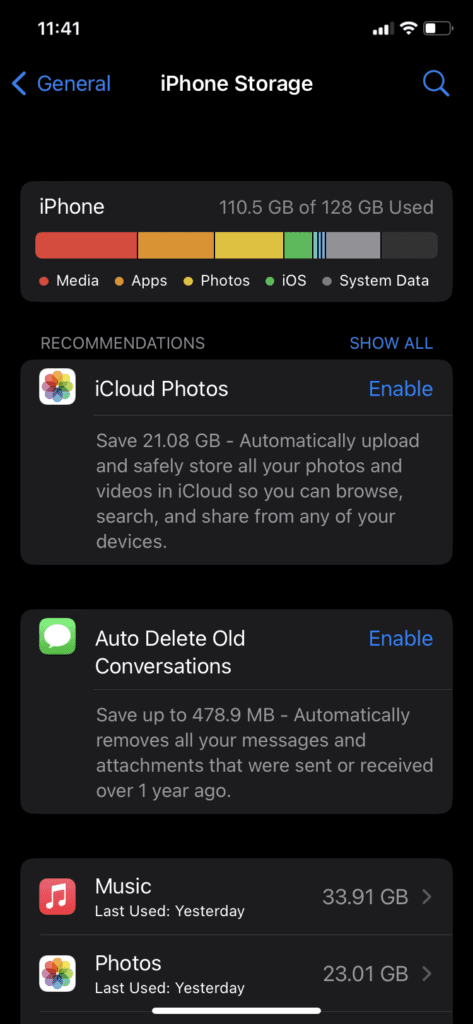This is an iPhone storage screen displayed in dark mode, with a black background and white text for clarity. At the top, the header reads "iPhone Storage" followed by the device name, "iPhone," showing that 110.5 GB out of 128 GB has been used. Below this, there is a tubular bar graph detailing the usage distribution among media, apps, photos, iOS, and system data.

Further down, there's a section labeled "Recommendations" with a "Show All" option in blue text on the right. The first recommendation suggests using iCloud Photos, which could save 21.08 GB by automatically uploading and storing all photos and videos in iCloud, allowing them to be accessed, searched, and shared from any device. The second recommendation is to auto-delete old conversations, potentially saving up to 478.9 MB by automatically removing messages and attachments older than a year.

Below the recommendations, there's a breakdown of specific storage usage: the Music app, last used yesterday, occupies 33.91 GB, while Photos, also last used yesterday, takes up 23.01 GB.